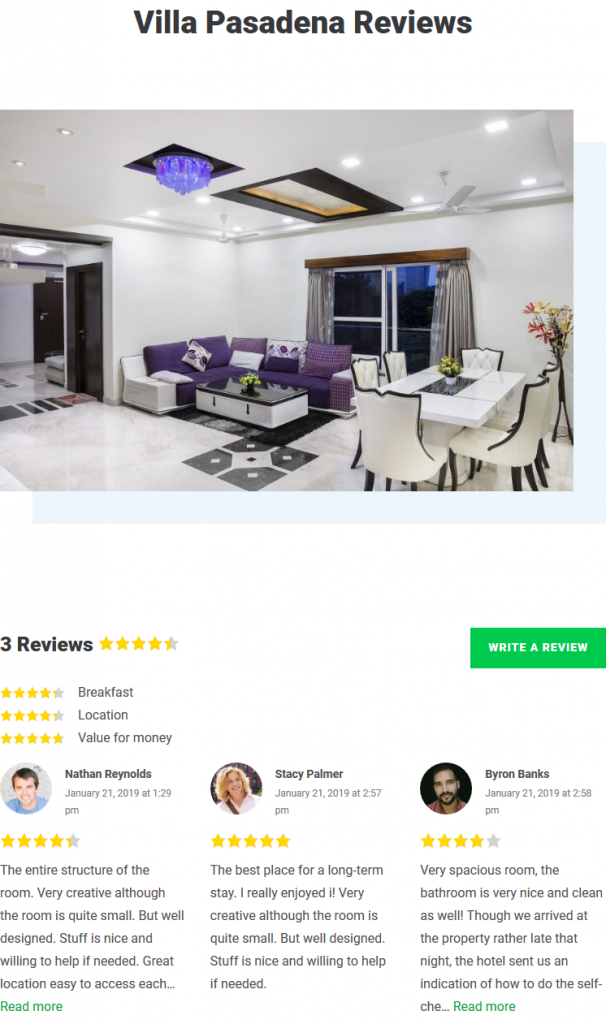**Detailed Descriptive Caption:**

The image showcases a screenshot from an unspecified website, topped by the header "Via Pasadena Reviews." The primary focus of the photograph is a sophisticatedly designed large white room, notable for its elegant, modern decor. Hanging prominently from the ceiling is a striking purple chandelier, joined by a ceiling fan and a skylight that likely fills the room with natural light during the day. The ceiling also features multiple areas of recessed lighting, enhancing the room's ambiance.

In the corner rests a luxurious couch, upholstered in a blend of purple and white. The couch is embellished with an assortment of matching purple and white throw pillows that enhance its visual appeal. Positioned in front of the couch is a sleek coffee table, finished in a contemporary black and white design.

An open window with the curtains pulled back suggests it is nighttime. To the right side of the room, a white dining table is surrounded by stylish white dining chairs that have black trim, creating a chic monochrome effect.

The website indicates that there are three reviews for this place, with an overall average rating of 3.5 out of 5 stars. In more specific ratings, breakfast received 4.5 stars, the location got 4 stars, and the value for money was awarded a perfect 5 stars.

- **Nathan Reynolds** (January 21st, 2019 at 1:29 PM, 4.5 stars): "The entire structure of the room is very creative although it is quite small but well-designed. The staff is nice and willing to help if needed. Great location. Need to access each... Read more."
  
- **Stacey Palmer** (January 21st, 2019 at 2:57 PM, 5 stars): "The best place for a long-term stay. I really enjoyed it. Very creative although the room is quite small but well-designed. The staff is nice and willing to help if needed."
  
- **Byron Banks** (January 21st, 2019 at 2:58 PM, 4 stars): "Very spacious room. The bathroom is very nice and clean as well. Though we arrived at the property rather late that night, the hotel provided us with detailed instructions for self-check-in.... Read more."